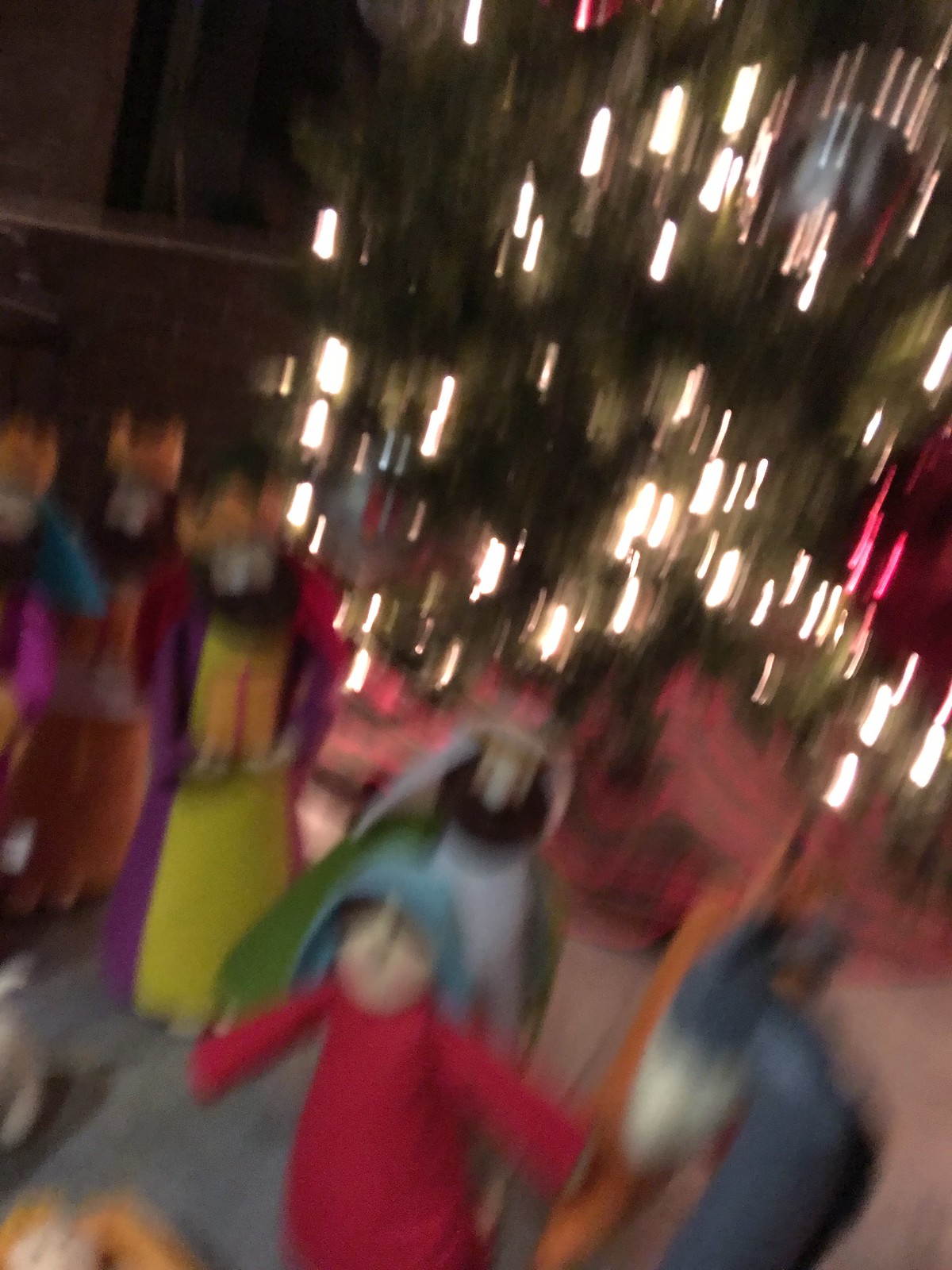This is a blurred photograph depicting a potential Christmas display. At the front, there appear to be three doll-like figures positioned as Joseph, Mary, and baby Jesus, based on traditional nativity arrangements. In the background, three other figures, possibly representing the Three Wise Men, stand solemnly. Soft, warm yellow lights twinkle in the backdrop, suggesting they may be part of a festive Christmas tree, although the image's blur makes it challenging to discern specifics with certainty.